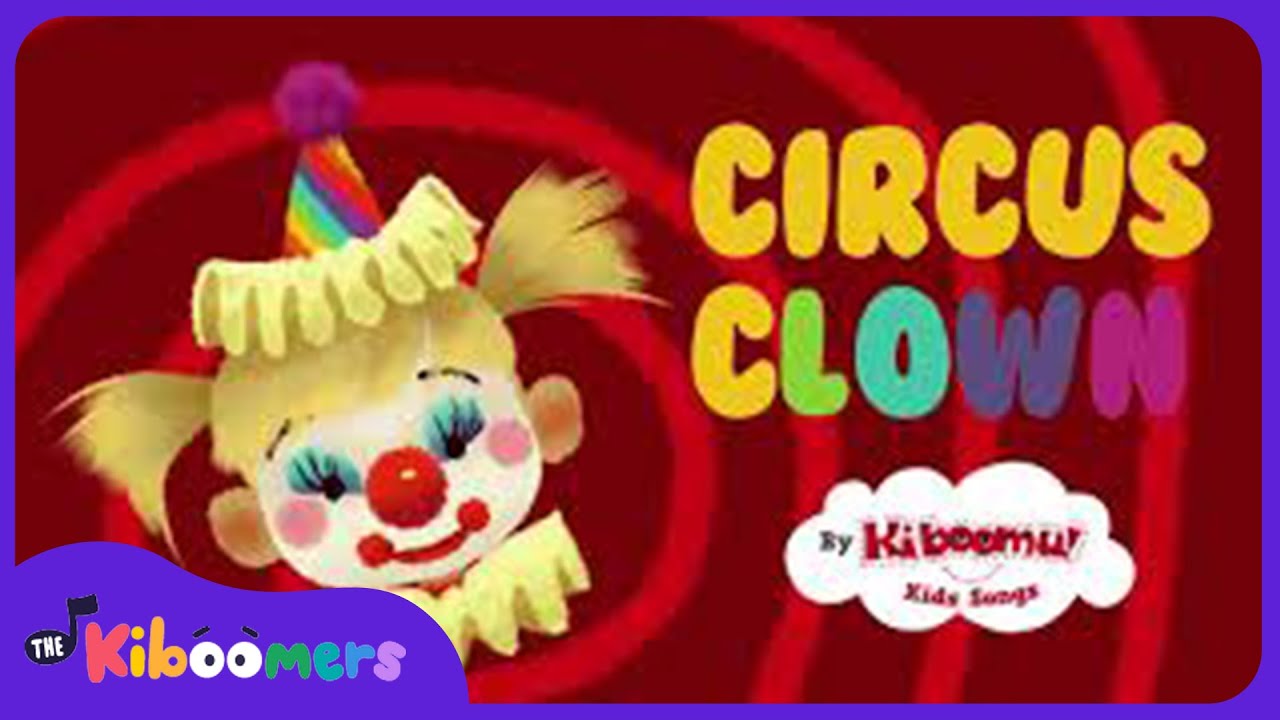The image is a vibrant and colorful advertisement, possibly for a children's television show or video thumbnail, featuring a little girl dressed as a clown. She has blonde hair styled into ponytails, sticking out from either side of her head, and is adorned with detailed clown makeup. Her face is painted white with red lips stretched into a wide smile, pink cheeks, a large red nose, and blue eye shadow accentuating her large eyelashes. She wears a rainbow-colored coned hat topped with a purple fuzzy ball, and yellow frills beneath the hat’s triangle portion. The background of the image features a swirling pattern of dark red and light red. On the right side of the image, colorful letters spell out "Circus Clown," with a thought bubble below that stating "by Kill Boomoo" and "Kid Songs." In the bottom left corner, the text reads "Kid Boomers." The overall illustration has a cartoonish and playful aesthetic, perfect for captivating a young audience.